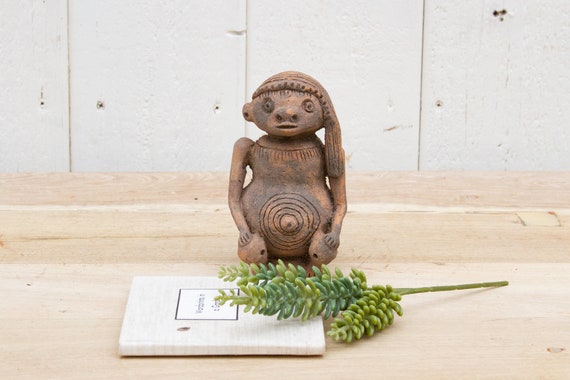This photograph captures an intriguing scene centered around a small, aged statue. The statue, which appears to be crafted from a dirty orange clay, bears a striking resemblance to a whimsical creature, perhaps reminiscent of ancient Incan artistry or a female troll character from popular media. The figure has a distinct headpiece or hair styled in a side part on the left, and a large swirly pattern decorates its belly, encircling a protruding belly button with multiple rings. This curious figurine, with expressive eyes, nose, and mouth, sits prominently on a light wooden countertop, creating a stark contrast against the white paneled background, which appears to be constructed from wood panels screwed together.

In front of the statue, there is a branch with green foliage sprouting small seeds in various shades of green. Beside the branch rests a white object—possibly a tile or a book—with an unreadable black square imprinted on it. The combination of these elements—the ancient-looking statue, the vibrant greenery, and the mysterious white object—together conjures an enigmatic and somewhat mystical tableau.